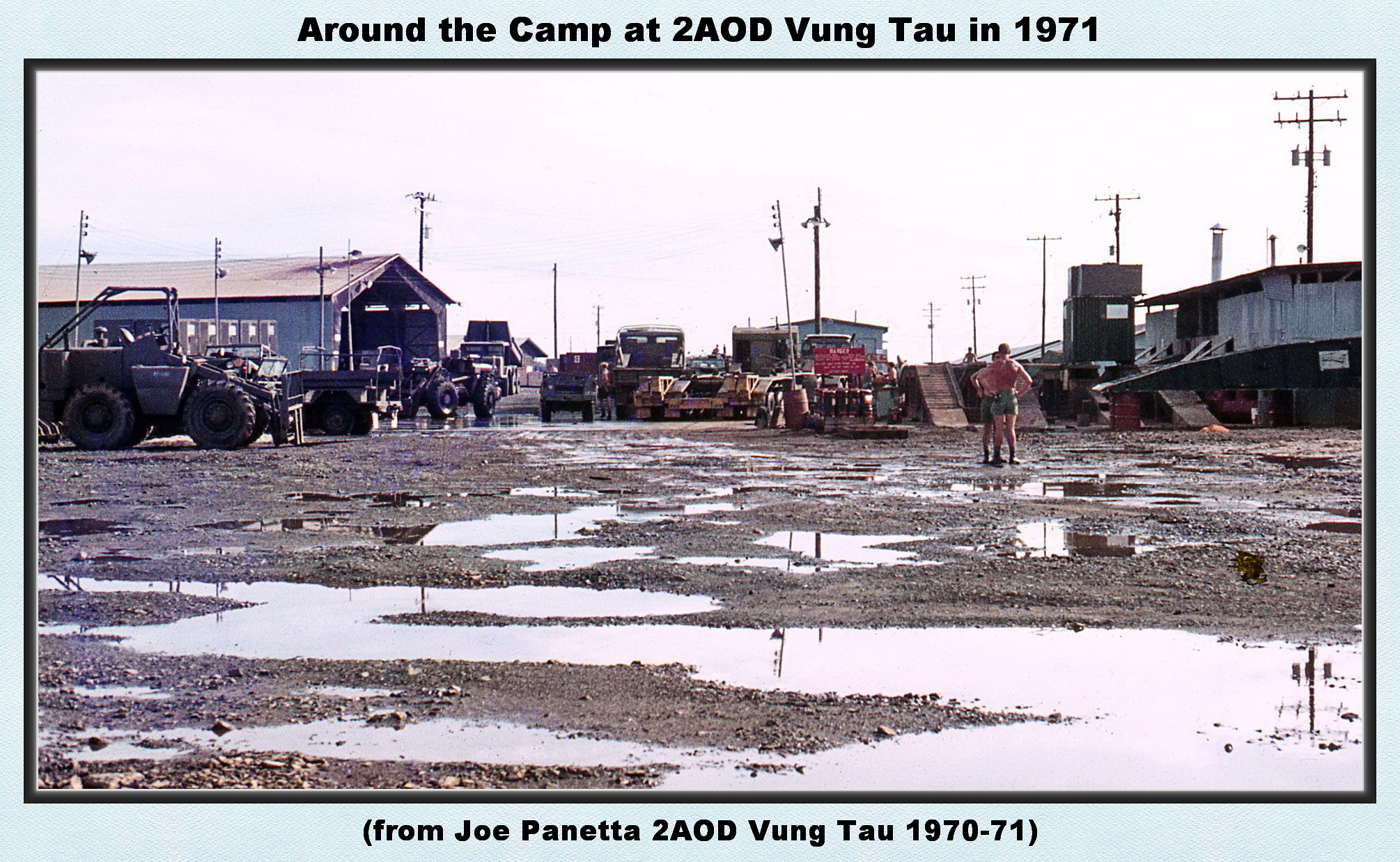This postcard-style image, framed with a light blue border, features black text at the top reading, "Around the Camp at 2AOD Vung Tau in 1971," and a caption at the bottom that states, "(From Joe Panetta 2AOD Vung Tau 1970 to 71)." The scene depicts a muddy, rocky ground with numerous puddles occupying the bottom half of the picture. The top half shows a military camp setting, characterized by a blue structure with a gray roof, possibly a large garage or hangar, and a variety of military vehicles, including jeeps with roll bars and trailers. Off to the right, another building is visible, and electrical poles dot the background. Two men, casually dressed in shorts with hands on hips, stand towards the back of the muddy field, adding a human element to the otherwise rugged and industrial environment. The image conveys a sense of daily life and operation within the camp, reflecting a moment in military history during the early 1970s.